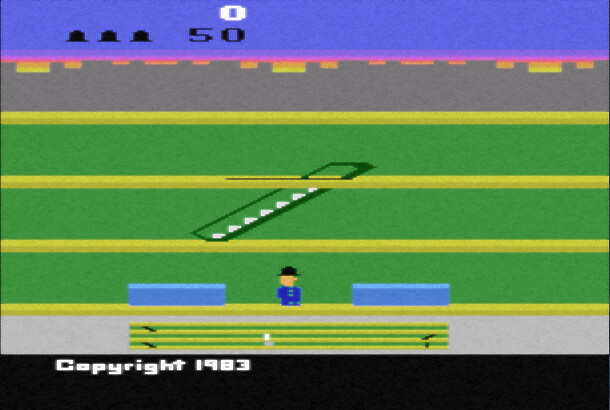This image appears to be a screen capture from an old video game, indicating a copyright of 1983 in white text on a black background at the bottom of the screen. The graphics are quite basic, indicative of early video game design. The lower portion of the screen features what seems to be green bleachers or a bench, resting on a silver path, suggesting the game's setting. A character, depicted as a male figure, stands in the middle wearing a blue coat and a black hat. This figure is flanked by two rectangular blue pillars. The game's environment is divided into multiple green lanes or paths, each separated by yellow lines. These lanes could represent different levels or segments the character must navigate. Above, a gray and blue outer line frames the screen, with three stem-like shapes possibly representing lives. Additionally, the number '50' is displayed, potentially indicating points or a score. The overall scene suggests a sports or track-and-field theme, intertwined with a multi-level gameplay structure.